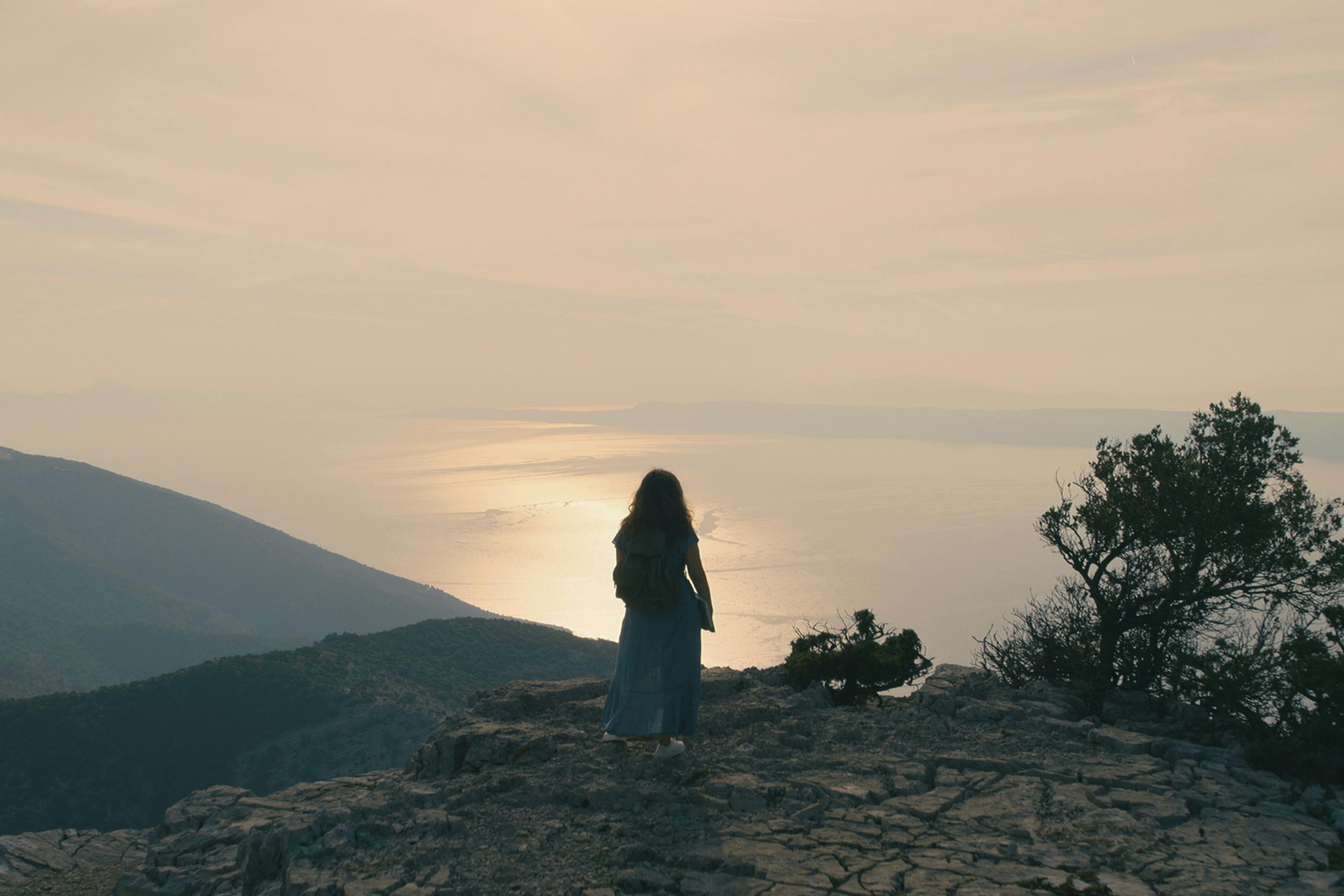A woman with long dark hair, dressed in a flowing blue dress and white tennis shoes, stands at the edge of a rocky, gray mountaintop, gazing out over a vast body of water that could be an ocean or lake. She has a backpack on her back and holds a book or journal in her right hand. The sun is setting, casting a twilight glow across the scene. To her left, distant hills and mountains rise up, while to her right, small bushes and trees frame the edge of the cliff. The water below reflects the sun's gleaming rays, adding to the serene beauty of the image. In the distance, a strip of land traces the horizon, partially shrouded in fog, with clouds adding texture to the sky. The woman's back is to the viewer, emphasizing her contemplative stance as she takes in the breathtaking natural landscape.